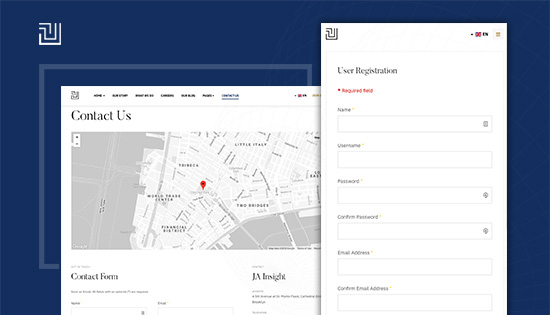This is a detailed screenshot of a registration screen from a web page or app, set against a dark blue background. In the top left corner of the screen, there is a logo, which consists of a square formed by intersecting lines. The main content of the screenshot is a light blue outlined box, positioned towards the left center of the screen. Overlaid on top of this outlined box is a contact page pop-up with a white background.

At the top left of this pop-up, large black letters spell out "Contact Us." Directly beneath this title is a large map centered within the pop-up. Below the map, the words "Contact Form" are displayed. To the right side of this pop-up is another section dedicated to user registration. This section has a large rectangular box with a white background and a similar square logo in the top left corner.

Within the registration section, there are fields for "Name," "Username," "Password," "Confirm Password," "Email Address," and "Confirm Email Address," each associated with corresponding text boxes for user input. No other identifying information is present in the screenshot apart from the logos.